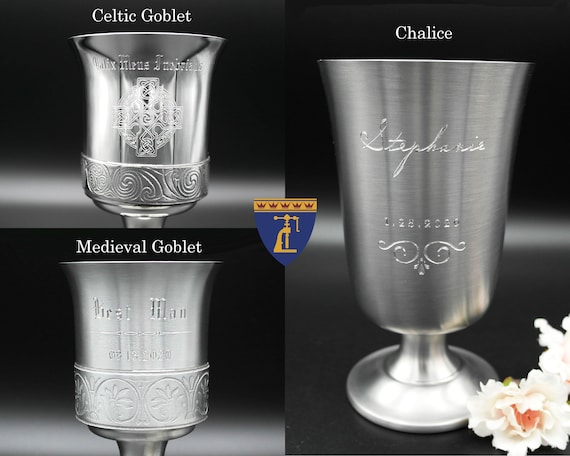The image presents a collage of three types of drinkware, all set against a dark background of black, dark gray, and white tones. At the top left is a shiny, silver-colored Celtic goblet with an inscription and white text above it reading "Celtic Goblet." Just below it is another bright silver goblet labeled "Medieval Goblet," which shares a similar design. Both goblets feature widened tops, narrow bottoms, and engraved details. Centrally positioned is a blue and yellow coat of arms insignia adorned with red accents. To the right is a larger silver chalice with intricate engravings, a very short stem, and an expanded base. Below the chalice, in the bottom right corner, are delicate white and peach-colored flowers, accompanied by white text stating "Chalice." Additional colors in the image include metallic silver, light green, blue, yellow, dark red, and black, creating a rich and detailed visual composition.